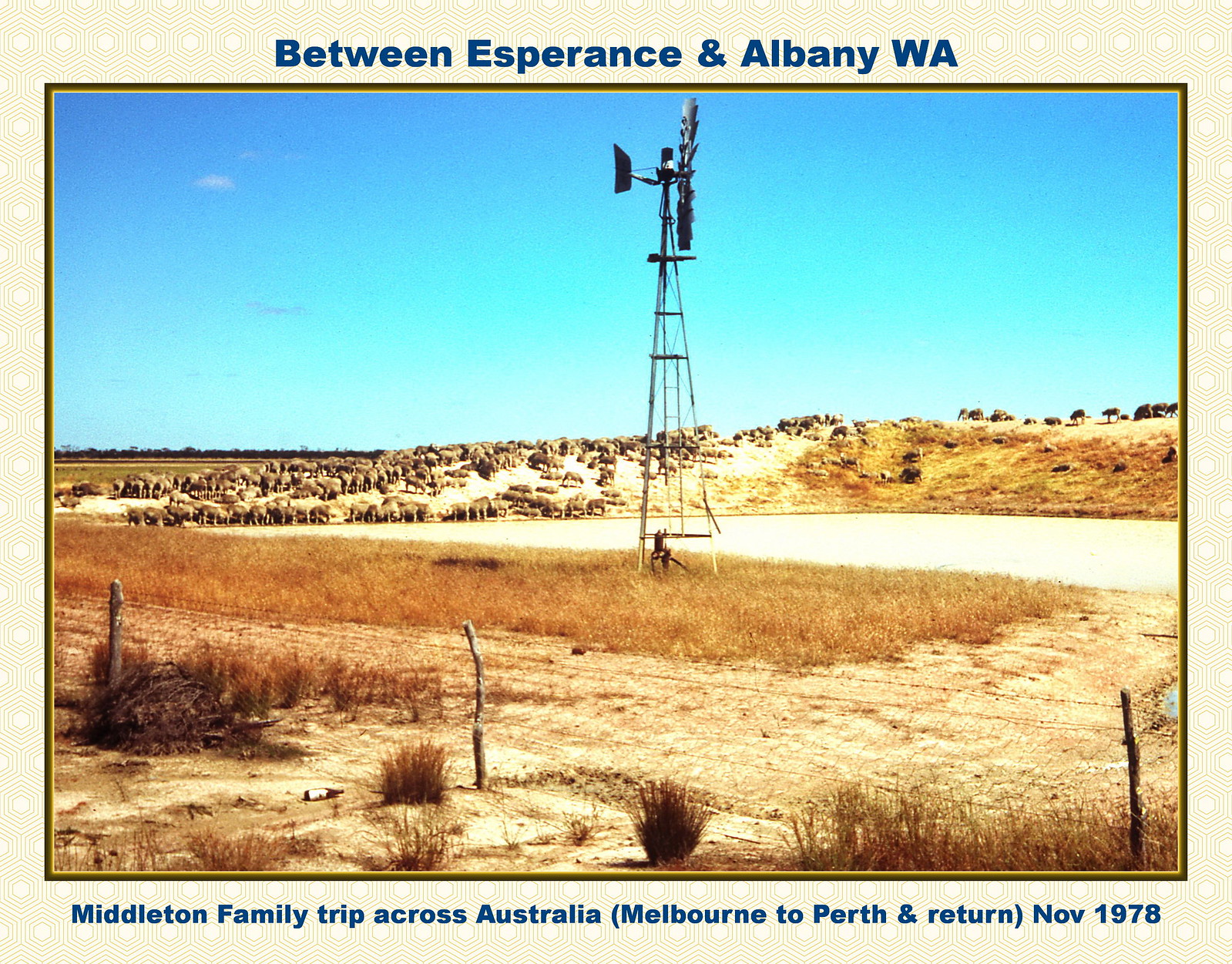This is a 1978 photograph capturing a pastoral scene between Esperance and Albany, WA, during the Middleton family trip across Australia, from Melbourne to Perth and back. The image is bordered with blue captions that read, "Between Esperance and Albany WA" at the top and "Middleton family trip across Australia, Melbourne to Perth and return, Nov 1978" at the bottom. The outdoor field depicted has areas of both green grass and barren ground. In the field's center stands a wind turbine, described as makeshift and somewhat rickety. Surrounding this turbine are various sheep grazing near an elevated patch of ground. The scene includes a faintly visible wired fence supported by visible wooden sticks, with an empty bottle lying in front. The sky above is clear and blue, creating a tranquil backdrop for this nostalgic family memory.